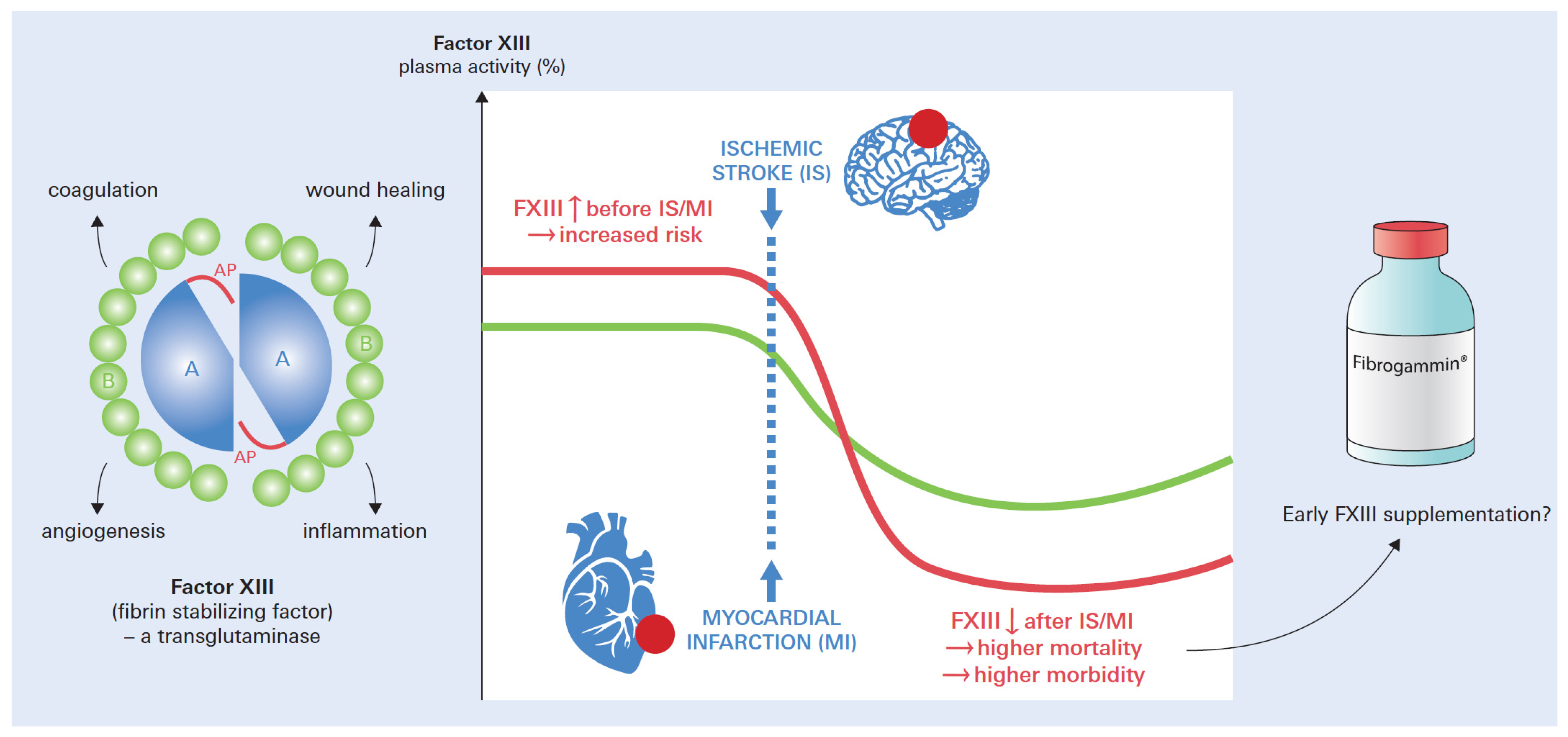The image depicted is a detailed cartoon infographic commonly found in scientific textbooks or displays, featuring a light blue background. On the right, there is a blue bottle with an orange lid labeled "Fibrogammon: Early FXIII Supplementation?" 

Central to the image, a white rectangular box showcases blue graphics of a brain at the top and a heart at the bottom, labeled "Ischemic Stroke" and "Myocardial Infarction (MI)" respectively. Red and green lines traverse the box, indicating different pathways and linking various medical conditions and risks such as increased risk, higher mortality, and higher morbidity. 

On the left side, a graphic illustration features Factor XIII, Fibrin Stabilizing Factor and Transglutaminase depicted with two blue segments of a circle connected by red lines and surrounded by green dots. Arrows emanate from the green dots towards labels like coagulation, wound healing, angiogenesis, and inflammation. This side also includes texts like "Factor XIII Plasma Activity Percentage," "Coagulation," "Wound Healing," "Angiogenesis," and "Inflammation."

The whole infographic centers on the complexities of ischemic stroke and myocardial infarction, highlighting the potential benefits and risks of early FXIII supplementation for these conditions.